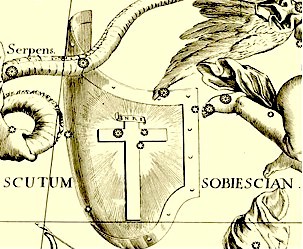The image presents an old piece of artwork dominated by a shield-like object at its center. The shield, slightly curved on the sides, prominently features a cross inscribed with the letters "INRI" at the top. Surrounding the central shield are various intricate details: on the bottom left, the word "Scutum" is visible, while on the bottom right, the term "SubYearScan" (or possibly "Sobeasian" as per the second description) is written. Additionally, to the upper left of the shield, there is a depiction of a partial snake, seemingly held by a hand, and labeled "Serpens." The top right corner reveals part of a bird's wing, partially obscured. The artwork is predominately yellowish to light brown in color, with the drawing rendered in different shades of brown. Vertical and horizontal lines extend from the top to the bottom and from left to right respectively, adding to the intricate composition of the piece.